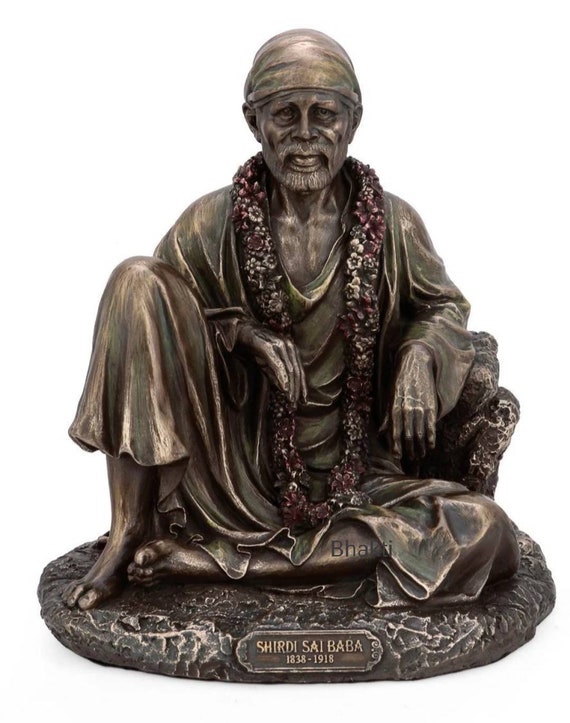The image is a detailed photograph of a statue depicting an old man, Shirdi Sai Baba (1838-1918), crafted from a dark metal with a brassy sheen. The figure is adorned with a mustache and beard, and his head is covered with a turban or scarf. He is dressed in loose-fitting robes and a prominent floral wreath that extends from his neck to his legs. The statue shows him seated on a circular, rocky plinth, barefoot, with one leg crossed and the other bent with the foot flat on the base. His arm rests casually, likely on a pillow or floor chair. The base of the statue includes a plaque inscribed with his name "Shirdi Sai Baba" and his years of birth and death. Notably, there is a faint gray watermark near his crossed leg that reads "BHAKTI," subtly blending with the statue's dark coloration. The background of the image is almost stark white, providing a striking contrast to the statue's muted tones.